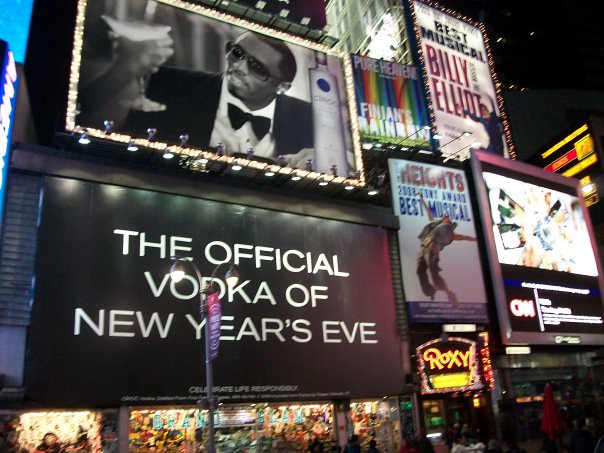The image showcases a vibrant scene filled with various signs and billboards, likely located in New York City's bustling Times Square. Dominating the scene is a large advertisement proclaiming, "The Official Vodka of New Year's Eve: Celebrate Life Responsibly," accompanied by a screen displaying a photograph that appears to feature Sammy Davis Jr. wearing sunglasses, with a hand holding up a glass in a toasting gesture.

To the right of this advertisement is a smaller sign labeled "Pure Heaven," next to another sign promoting the musical "Finian's Rainbow," adorned with rainbow colors. Adjacent to these, another sign celebrates the musical "Billy Elliot," depicting a man dancing on the lower right side of the billboard. Below this, another sign references "Heights," mentioning a Tony Award for Best Musical, though the fine details are blurred and unreadable.

Additionally, a corner of the image features a screen with the "CNN" logo at the bottom left. Beneath the "Heights" billboard, there's a sign for "Roxy," displayed in gold lettering with colorful lights encircling it. The scene is electrifying and chaotic, a testament to the dynamic energy of one of New York City's most iconic locations. The lower parts of the photo, especially under the vodka sign, are less discernible, adding to the bustling and overloaded sensory experience of the area.